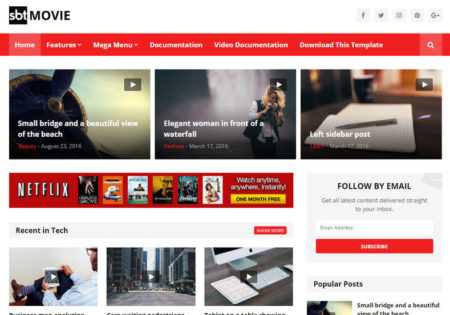The image shows a screenshot from the SBT Movie website, resembling a Netflix-like streaming platform. At the top of the site, there is a prominent red navigation bar that stretches across the entire width, containing several menu options: Home, Features, Mega Venue, Documentation, Video Documentation, and Download This Template.

Below the navigation bar, the website showcases a selection of movie thumbnails available for viewing. The first movie listed is titled "Small Bridge and a Beautiful View of the Beach." The second movie is "Elegant Woman in Front of a Waterfall," followed by one labeled "Left Sidebar Post." 

Further down the page, there’s a Netflix advertisement featuring six videos. The ad promotes Netflix's service with the tagline "Watch Anytime, Anywhere Instantly," and includes a yellow call-to-action button offering "One Month Free."

Additionally, the page includes an email subscription section labeled "Follow by Email," with a field for entering an email address and a red "Subscribe" button.

Towards the lower part of the page, there are three more video thumbnails, although their titles are not fully visible due to the way the image is captured. In the bottom right corner, there is a section labeled "Popular Post," which appears to be another clickable area for navigating the site's content.